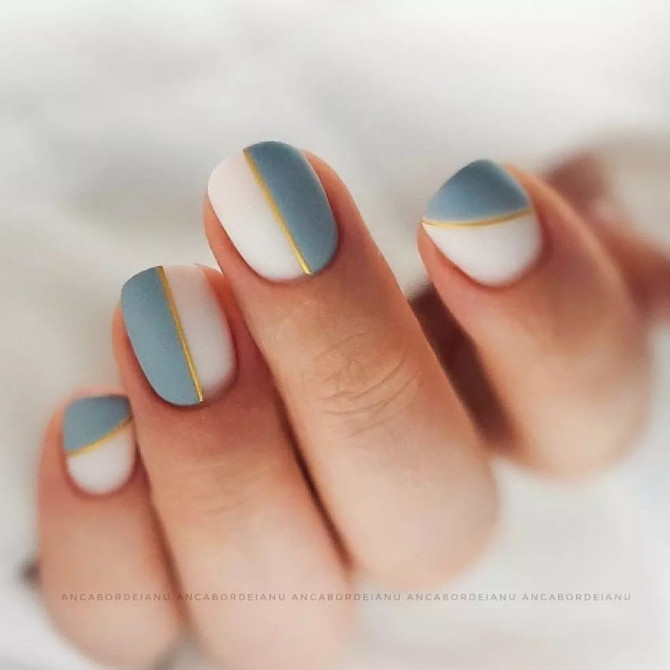The photograph showcases a close-up of a woman's hand lying on its side, with white blurred background. The focus is on four fingers - the thumb is out of focus and not visible. The fingernails are elegantly painted with a combination of white, bluish-gray, and gold. The index and pinky fingers feature a thin, curved gold stripe that runs diagonally, creating a white section at the bottom and a bluish-gray section at the top. The middle and ring fingers display a vertical gold stripe running straight down the center. The middle finger has a white section on the left and a bluish-gray section on the right, while the ring finger's color sections are inversed, with bluish-gray on the left and white on the right. The entirety of the photograph is overlaid with a watermark, "Anca Bordeianu," repeated several times near the bottom of the image.